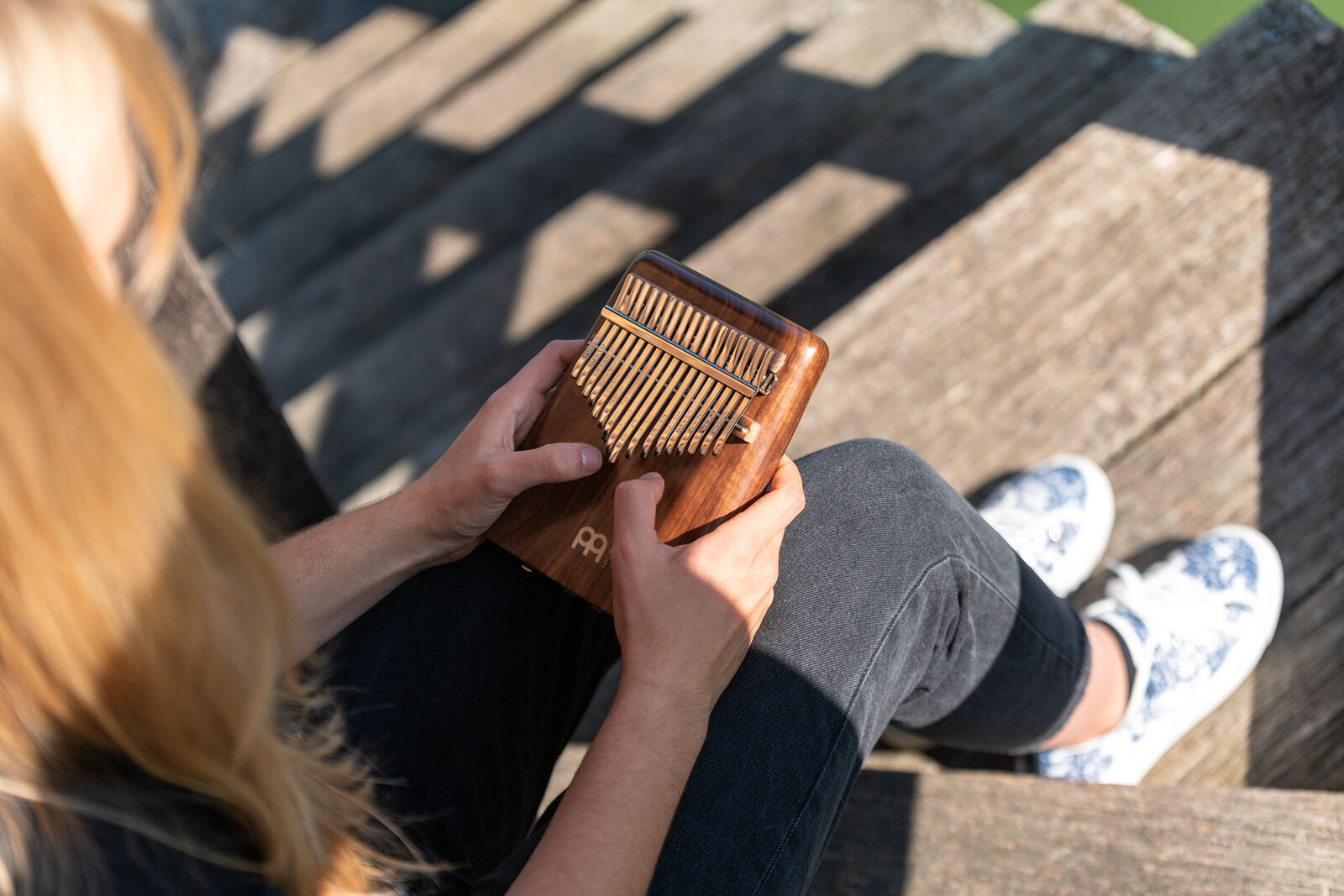The image captures an outdoor scene during the daytime, with sunlight illuminating wooden steps and casting shadows of the railing. Seated on these steps is an older white woman, possibly in her 40s or 50s, with long reddish-blonde hair accented by gray near her bangs. The photo is taken from above, looking down over her shoulder, so her face is obscured by her hair. She is wearing black jeans and striking blue canvas shoes adorned with white details and white laces, with her ankles exposed.

In her hands, she holds a small wooden instrument featuring copper or golden bars, arranged vertically and secured by a horizontal bar, resembling a miniature xylophone or micro-instrument with chimes. The instrument, which she plucks to produce sound, rests on her lap as she sits on the steps. The scene, illuminated by the sun shining from behind her, captures the serene moment with detailed emphasis on her attire and the unique instrument she holds.